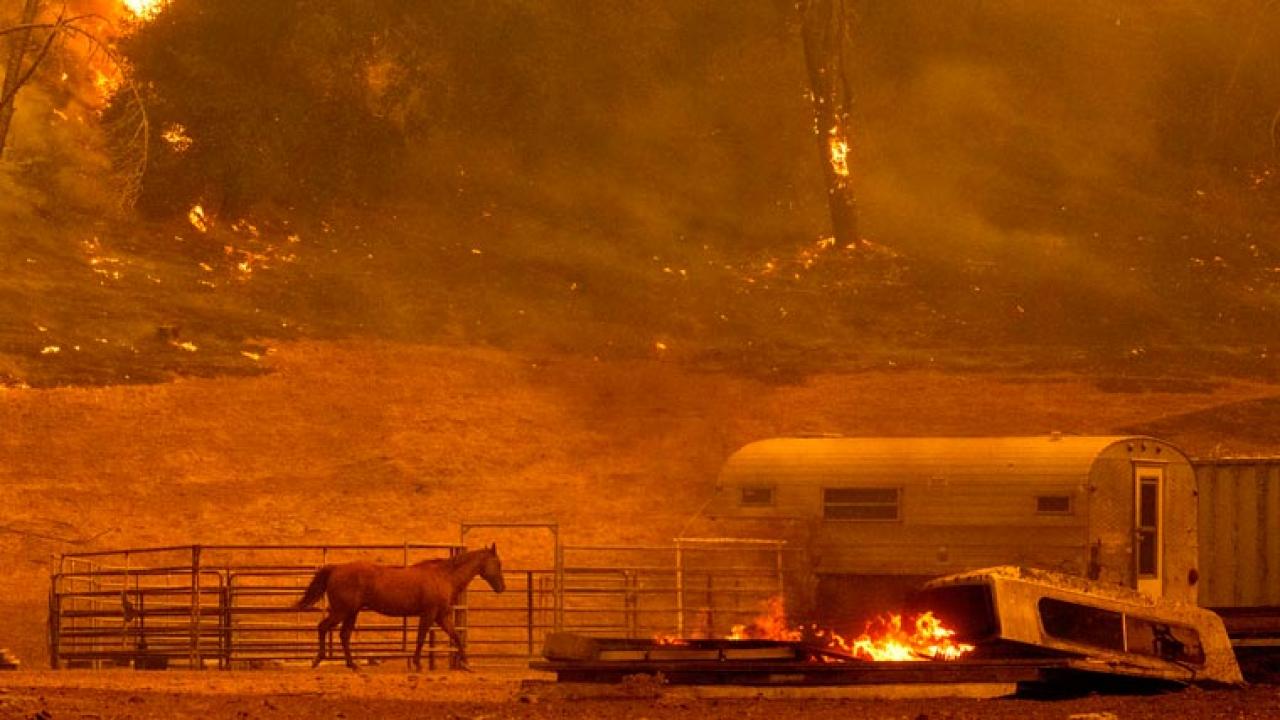The photograph captures a harrowing scene of a wildfire engulfing a rural area, painting the entire landscape in intense hues of orange and dark red. In the foreground, a solitary brown horse is either entering or walking past a metal gate, seemingly bewildered by the chaos around it. The gated area is flanked by a small camper building on the right and another nearby structure, possibly a shed. A camper shell lies on the ground with flames licking beneath it, adjacent to what appears to be a pile of metal debris. Bright yellow embers are scattered across the image, enhancing the fiery glow. In the background, smoke billows thickly, shrouding the sky and intensifying the dark, ominous orange tint. Disturbingly, a tree ablaze stands prominent in the distance, with additional smaller fires peppering the grassy terrain, particularly along the top left and upper center of the image. This heart-wrenching moment illustrates the relentless advance of the fire, which has consumed both the natural landscape and human-made structures, leaving the horse adrift in the midst of destruction.